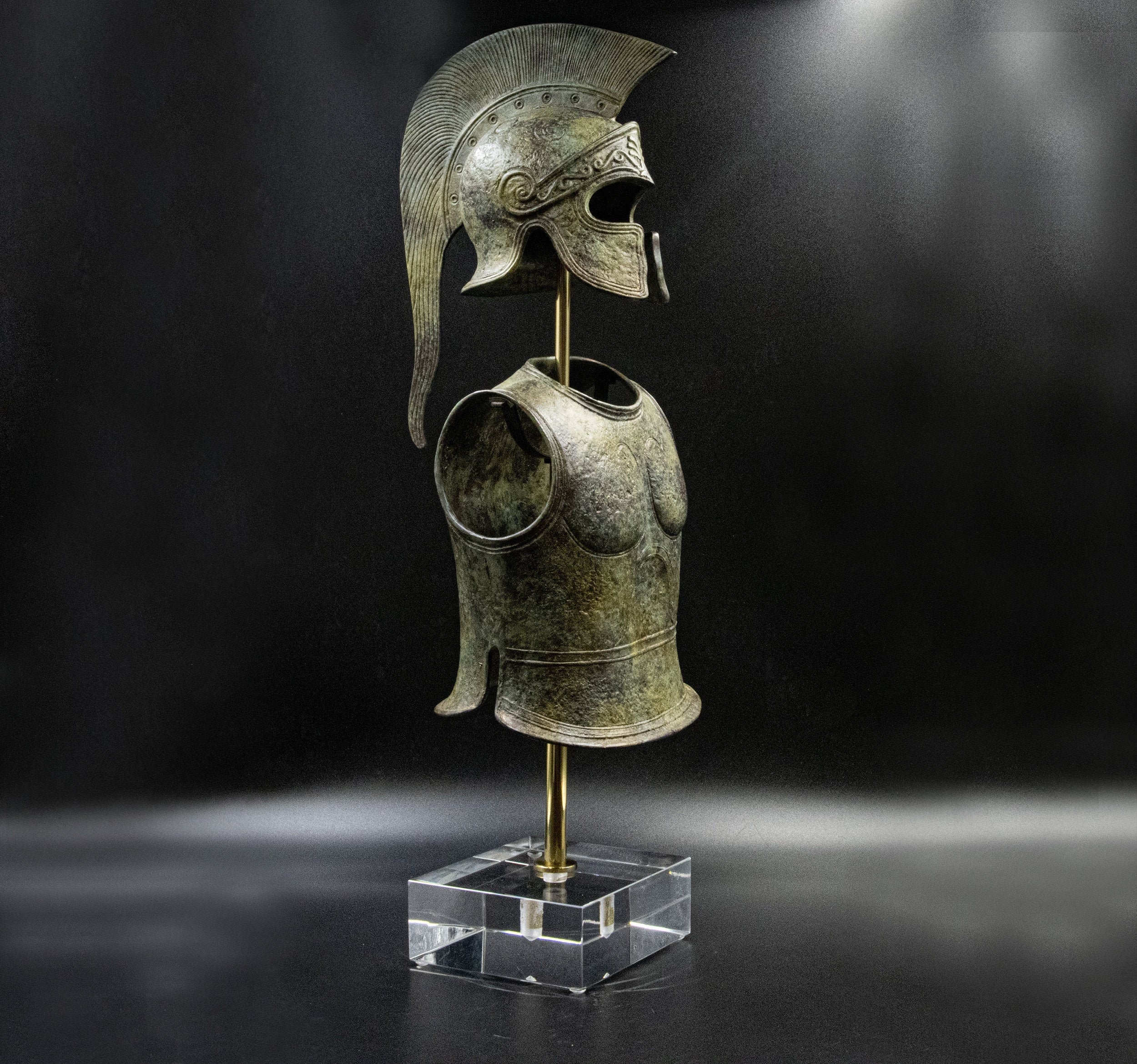The image depicts a detailed and intricately crafted miniature display of ancient Roman or Spartan warrior armor. Centered in the image, elevated on a brass-colored rod, is a tarnished, bronze chest plate exhibiting a greenish-black patina indicative of aged metal. The chest plate is designed without arms, showcasing openings for the head, arms, and legs. Above the chest plate, there is a helmet featuring a distinctive crest that tapers to a point, with slits for the eyes and mouth, forming a T-shaped opening. This ensemble is supported by a clear, crystal-like cubic base that sits on a table with a blurry surface. The whole setup is framed against a deep black background, adding a stark contrast and highlighting the historical and ornate details of the armor. The image gives the impression of a museum exhibit, meticulously displaying the iconic elements of a formidable ancient warrior.